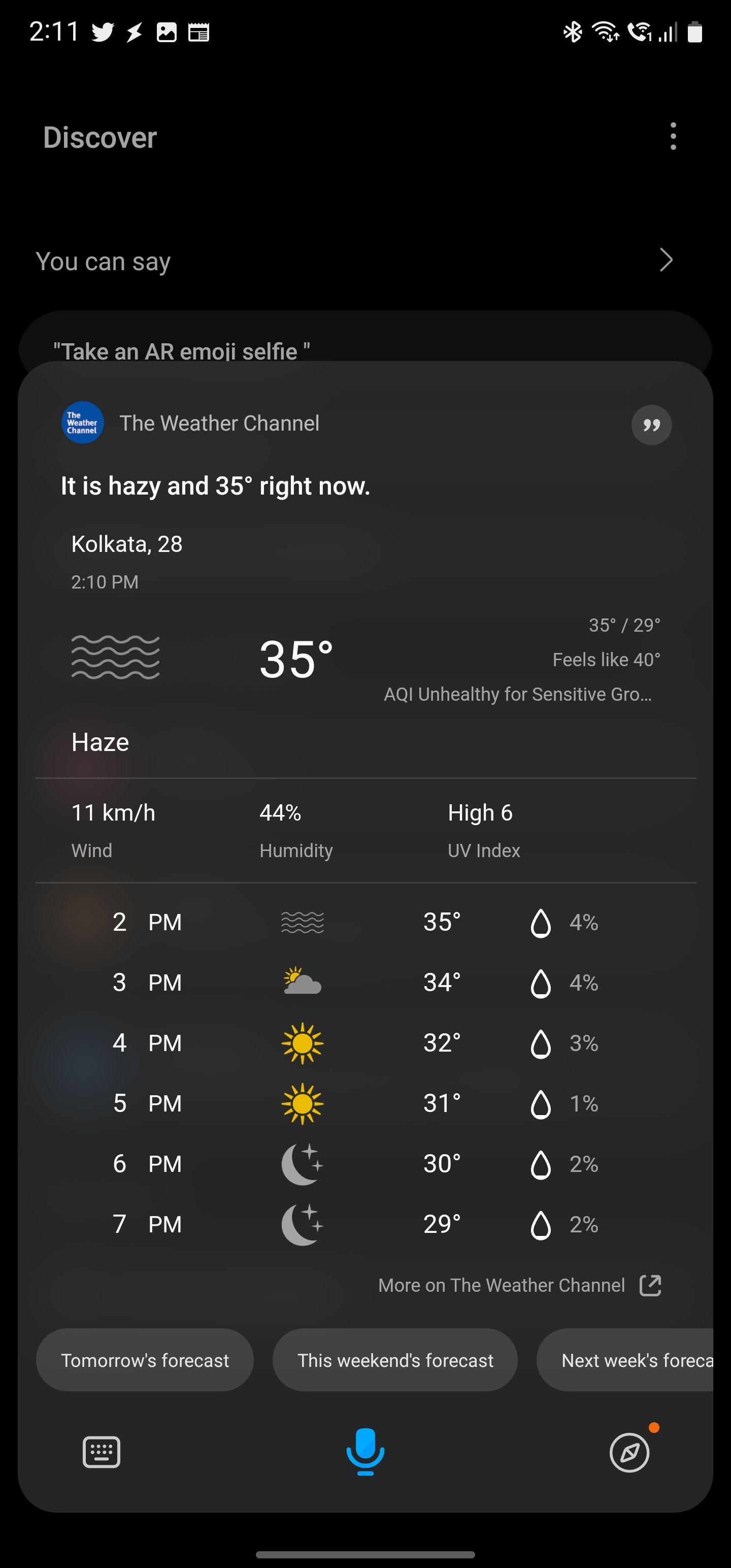A close-up view of an Android mobile phone screen displaying the Weather Channel app. At the top of the screen, a sequence of icons appears: the "2-11" timestamp, the Twitter icon, a lightning bolt, an image symbol, and a window or calendar symbol. On the right side, the status bar shows a Bluetooth symbol, Wi-Fi symbol, phone signal strength, and a battery symbol indicating 90% charge. The screen reads "Discover" in light gray letters, accompanied by a three-dot menu icon. Below, it prompts, "You can say," followed by a right arrow and the phrase "take an AR emoji selfie" in quotes.

An overlay with the Weather Channel logo reports "Hazy and 35 degrees" for Kolkata at 2:10 PM. The screen displays a "feels like" temperature of 40 degrees with an Air Quality Index (AQI) of "Unhealthy for Sensitive Groups." The term "Haze" is highlighted beneath this data. 

A gray line border separates additional weather information: "11 km/h wind," "44% humidity," and "high UV index of 6" are indicated. A detailed hourly table follows, listing temperature projections: 
- 2 PM: 35°C
- 3 PM: 34°C
- 4 PM: 32°C
- 5 PM: 31°C
- 6 PM: 30°C
- 7 PM: 29°C 

The detailed view effectively conveys current weather conditions and short-term forecasts for the user.